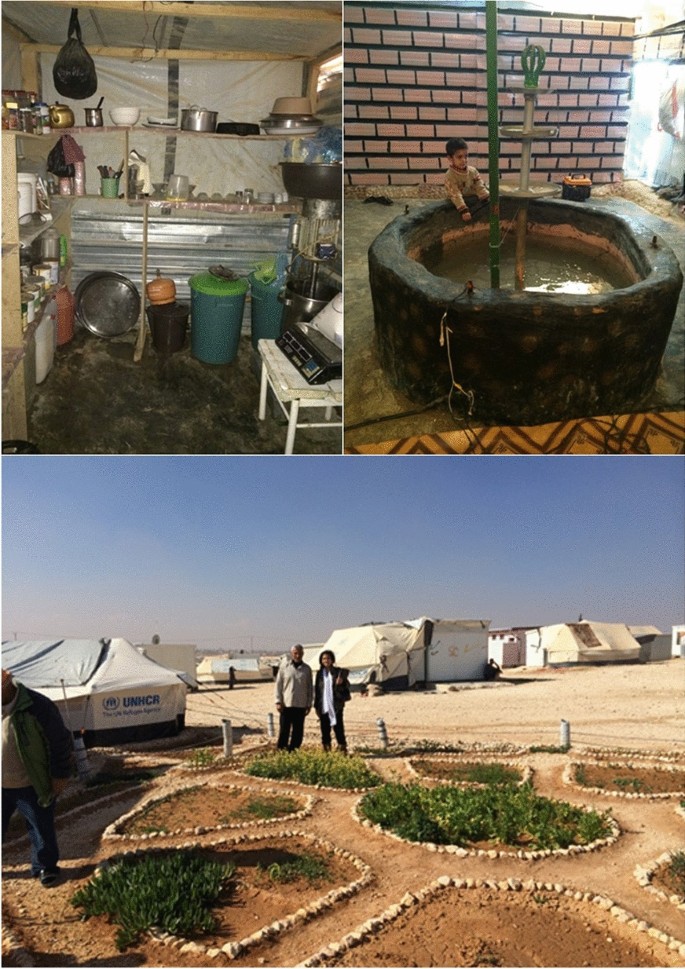The photograph is a collage of three distinct images, each depicting elements of what appears to be a humanitarian relief camp. The top left image captures the inside of a makeshift kitchen tent, reminiscent of those set up during group camping trips. It features a collection of old, tin-like pots, pans, and other cooking utensils, suggesting a rudimentary setting typical of a resource-limited environment.

The top right image showcases a rudimentary outdoor spa or hot tub made from natural stone, partially filled with water, and constructed within a brick-enclosed area. A young boy is seen standing beside the spa, interacting with the water, and adding a poignant human element to the scene.

The bottom image, which dominates the lower section of the collage, portrays two individuals standing in a vast field surrounded by numerous white tents, indicative of a temporary settlement. The individuals are dressed in jackets, and there are other people visible in the background, alluding to a busy camp environment. The tents bear symbols of a non-profit organization, akin to UNICEF, suggesting that the entire setting is part of a disaster relief effort aimed at assisting those in need.